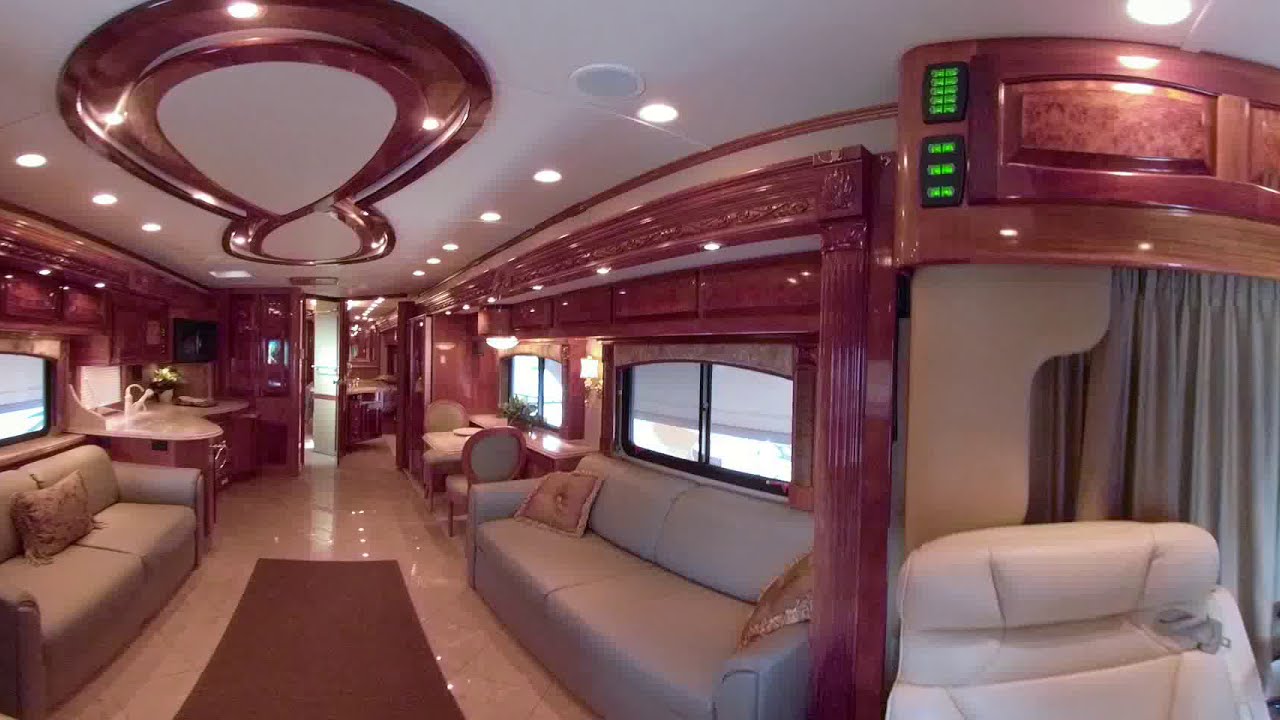This is an interior photograph of a luxury RV, showcasing an elegant and sophisticated design. At the front right corner, a plush, white leather driving chair is situated below a gray curtain with storage compartments and electronic control buttons above it. The floor is a light brown tile, polished to a shine, contrasting beautifully with a dark brown, round carpet in the middle. The RV features two cream-colored sofas, one larger than the other, flanking the narrow space, providing ample seating.

Above the sofas, there are numerous shiny mahogany storage cabinets with intricate carvings, reflecting the upscale finish. The ceiling is adorned with a figure-eight infinity wooden design in shiny mahogany, housing circular, white lights that illuminate the entire area. Windows line the walls, bordered by a subtle, dark pink design, allowing natural light to filter in and complement the indoor lighting.

Further into the RV, the kitchen area showcases a luxurious marble countertop, while the dining nook offers a cozy booth seating arrangement. Continuing towards the rear, there's a bathroom and a bedroom, completing the high-end, spacious layout of this opulent mobile home. The overall color scheme blends rich mahogany, cream, and mauve, enhancing the luxurious ambiance and making this RV a true mobile sanctuary.